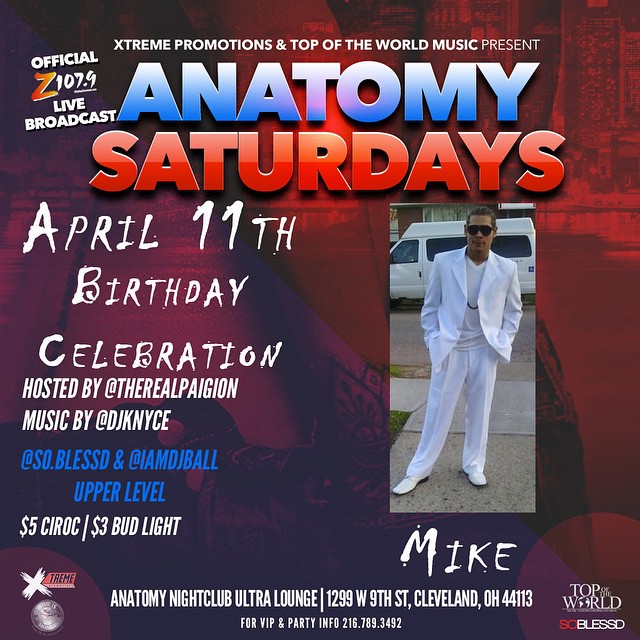The advertisement image features a vibrant, triangle-themed background with red on top and purple on the bottom. At the top left corner, in a smaller font, the text reads, "Extreme Promotions and Top of the World Music Present." Below that, the main event title "Anatomy Saturdays" is prominently displayed, with "Anatomy" in blue and white font outlined in black, and "Saturdays" in varying shades of red with a black trim. To the left of the main title, "Official Z 107.9 Live Broadcast" is noted, with the "Z" highlighted in a reddish-orange color. 

Further details on the left side include "April 11th Birthday Celebration" in white font, followed by "Hosted by @theRealPagon." Below, it mentions, "Music by @DJKNyce, @SoBlessed, and @IMDJBALL," with "Upper Level" in blue font. Promotional offers such as "$5 Ciroc" and "$3 Bud Light" are also listed in white font. 

On the bottom left, there is an emblem associated with "Extreme," alongside a photograph of a man in a white suit and dark shades standing by a white van on a sidewalk. The name "Mike" appears in white font beneath the photo. 

Centered at the bottom of the ad, the text reads, "Anatomy Nightclub Ultra Lounge," along with the address "1299 West 9th Street, Cleveland, Ohio 44113." Additional details concerning "Top of the World S.C." and "Blessed" are found in the lower right corner.